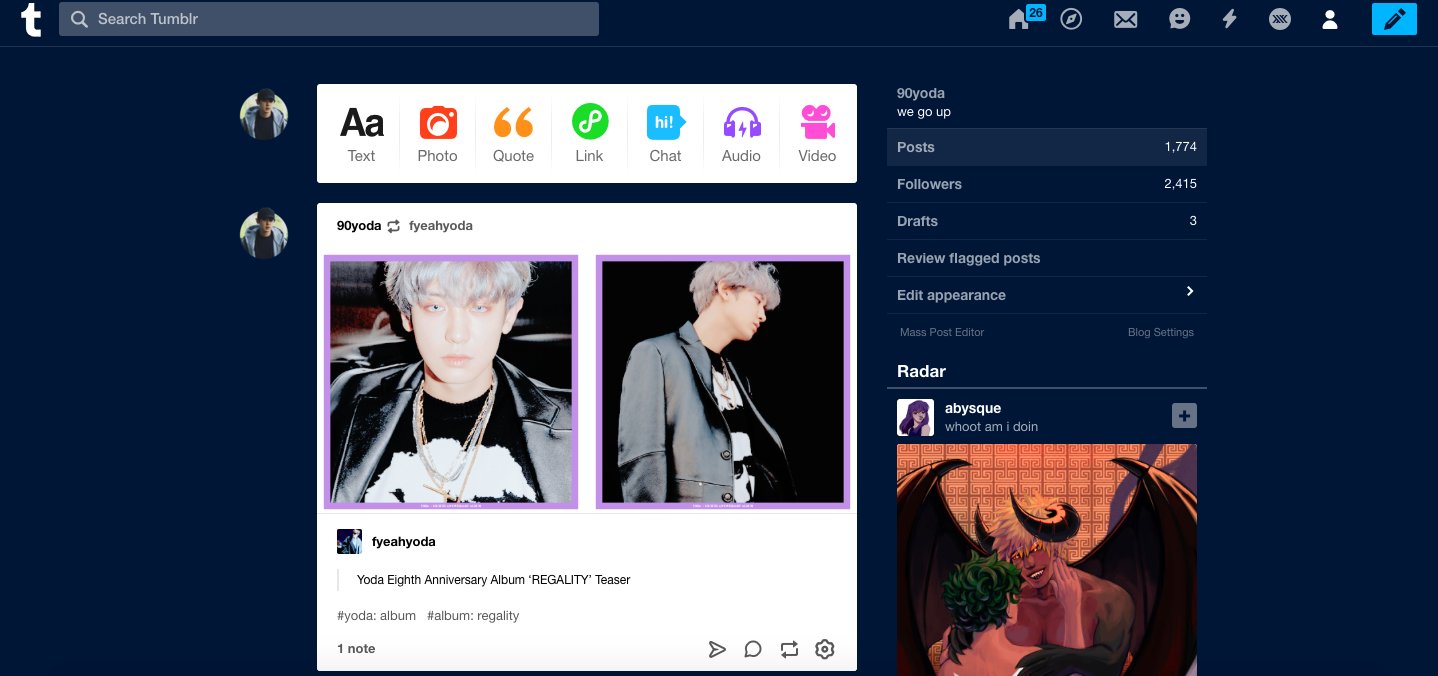This image captures a partial view of a Tumblr web page interface, filled with various icons and user-generated content. At the top left of the page, the familiar Tumblr logo is prominently displayed, followed by a search bar labeled "Search Tumblr." Adjacent to the search bar is a row of navigation icons: a home icon with the number 26 beside it, an unidentified circle icon, a male user icon, a smiling face emoji, a lightning bolt, a keyboard, a user profile icon, and a pencil icon.

Beneath this navigation bar, the main body of the page showcases a user’s profile photograph, flanked by a multi-tabbed content creation box labeled "AA Text," "Photo," "Quote," "Link," "Chat," "Audio," and "Video." Below this content box are photographs and posts related to "90 Yoda," a K-pop star celebrating his 8th anniversary, accompanied by a "Regality Teaser." The post has received one note and is followed by interactive icons for sending, chatting, refreshing, and changing settings.

Further down on the page, more details about the "90 Yoda" profile are displayed. The information includes post count (1,774), follower count (1,774), the years 2014-2015, the number of drafts (3), and options to review flagged posts or edit appearance, indicated by a right-facing arrow.

Additionally, there is a "Radar" section which highlights a user named "Abby-esque" with a tagline that reads, "What am I doing?" Below this are images of an animated couple, featuring a gargoyle and a woman, giving the page a touch of whimsical storytelling.